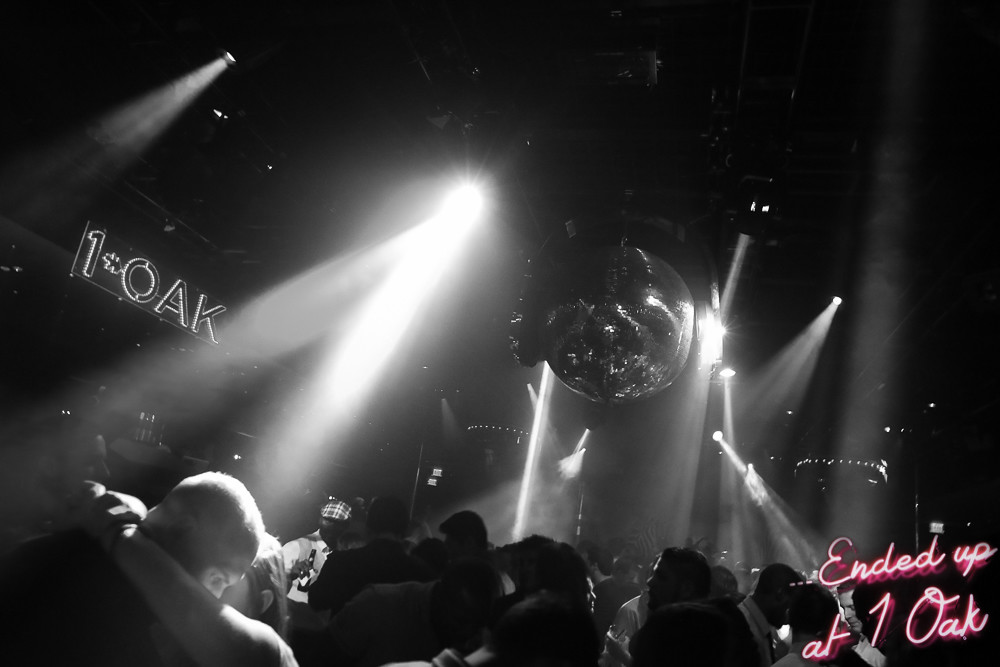The black-and-white photograph captures a lively scene inside a nightclub, most likely One Oak, as indicated by a logo on the left side of the image. Bright, laser beam-style spotlights illuminate the otherwise dark room, streaking down from the ceiling. A large, unlit crystal ball hangs prominently overhead. The foreground is bustling with people dancing and socializing, with a couple on the left engaging in a public display of affection; the woman has her arms around the man's neck. The composition focuses upwards towards the ceiling, capturing the energetic atmosphere of the venue. At the bottom right corner of the photo, text in pink neon-style letters stands out, reading "Ended Up at One Oak," adding the only touch of color to the monochromatic scene.